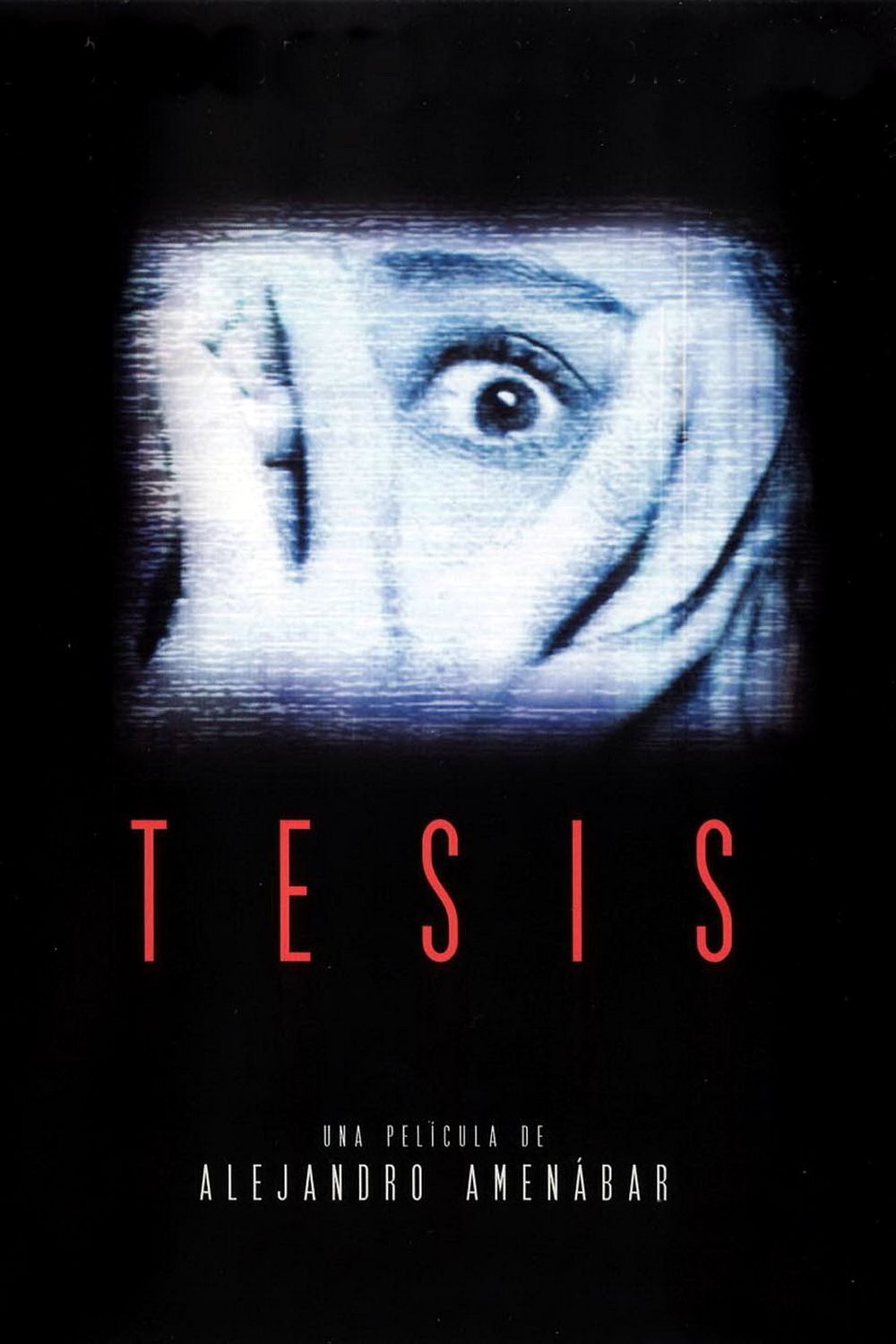This is a movie poster with a stark black background. Dominating the center is a blurry, static-like image of a face mostly covered by hands, creating a vertical rectangular focal point. The hands are positioned such that two fingers are to the left and two to the right of a single visible eye, which is wide open and appears scared. The face, likely of a Caucasian individual, has short black eyelashes and a visible eyebrow, adding to the intensity of the gaze. Below this haunting image is the movie title, "T-E-S-I-S," written in bold red letters. Further down, in smaller white text, are the words "Una película de Alejandro Amenábar," indicating the film's director.